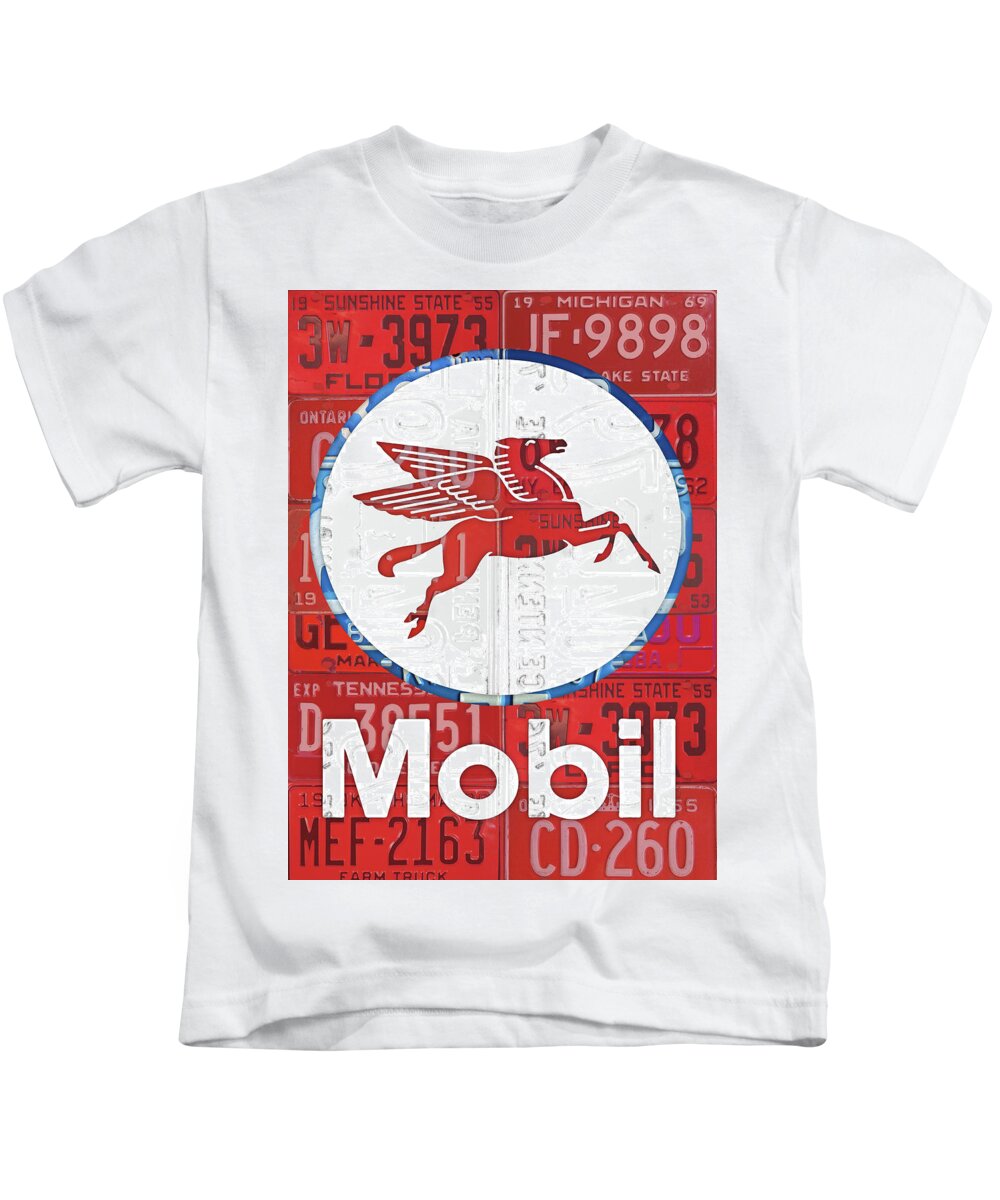This is a full-color photograph of a white short-sleeved t-shirt laid flat on a plain white surface, with its slightly wrinkled fabric indicating it has not been smoothed down. The t-shirt features a vertically rectangular red graphic prominently displayed on the front. This graphic contains a colorful collage of old license plate designs from various states and regions, including readable plates like those from Florida, Michigan, Tennessee, and Ontario. Superimposed on these plates, a bold white section at the bottom of the graphic displays the word "Mobil" in large letters, an unmistakable reference to Mobil Oil. Above this text, in the middle of the graphic, there is a white circle with blue trim, featuring the iconic red Pegasus logo of Mobil, with the horse flying to the left. The high level of detail in the design reflects a vintage, nostalgic theme, making the t-shirt intriguing and unique.